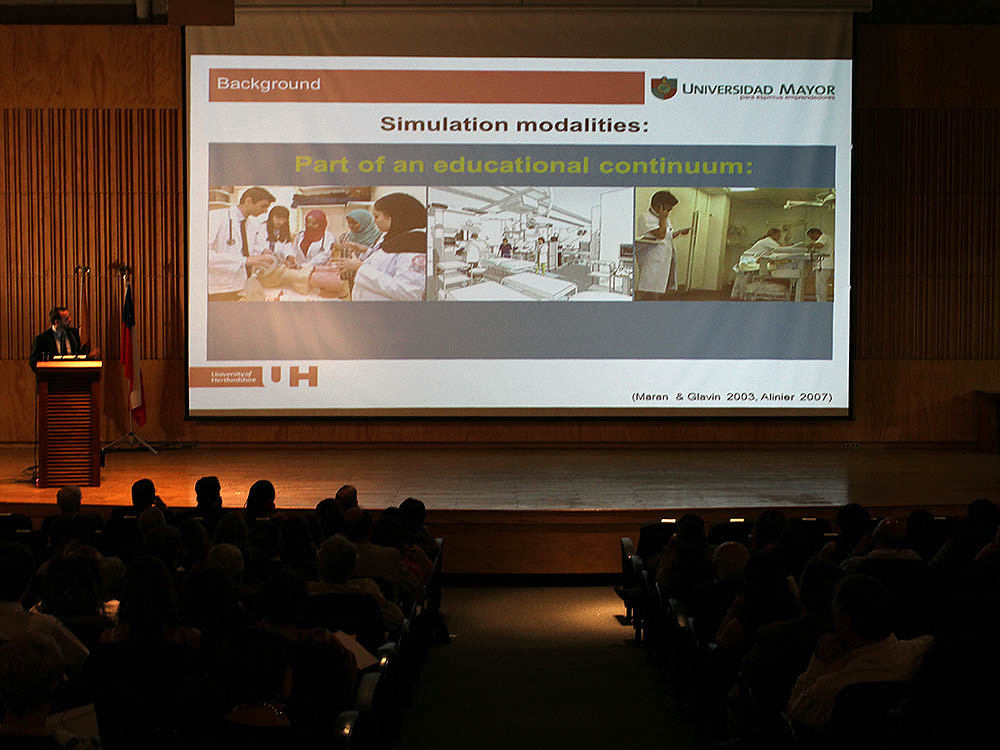This is a detailed color photograph in landscape orientation, capturing an interior setting of a convention hall. The scene features a stage at the foreground with a darkened audience viewing the presentation. The audience is silhouetted, revealing only the backs of their heads. On the left side of the stage stands a man at a wooden podium, dressed in a suit and tie, with a flag behind him. He is intently looking at a large, illuminated projection screen situated at the center of the stage.

The projection screen displays a detailed slide with a distinctive red strip at the top bearing the white letters "background," accompanied by the logo of Universidad Mayor. The slide title reads "Simulation Modalities" with the subtitle "Part of an educational continuum" in yellow text on a gray background. The slide includes three color photographs, depicting scenes of medical practice: one shows nursing students working on a mannequin head, the middle one illustrates a hospital room, and the rightmost image features a scene in what appears to be a hospital or dental office. The bottom of the slide displays the dates "2003" and "2007." The surrounding environment carries a burgundy hue, enhancing the ambiance of a formal educational presentation.